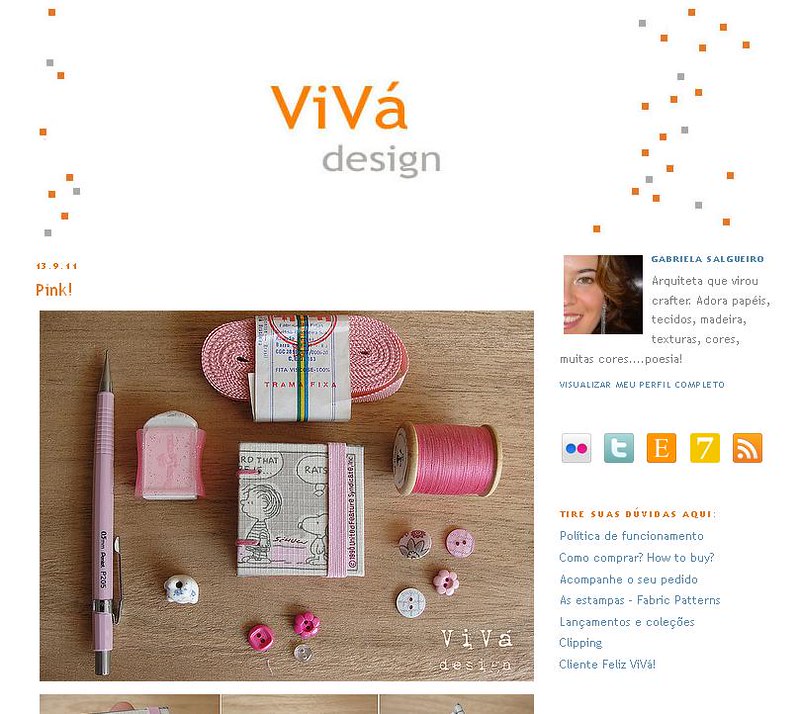The image appears to be a webpage with a white background featuring vibrant elements in orange and gray. At the top, "VIVA" is prominently displayed in bold orange text, followed by "design" in gray underneath. Below this heading is a visually cohesive display of various pink items arranged on a brown wooden table, including a mechanical pencil, an eraser, a spool of thread, several buttons, and shoelaces. Central to this arrangement is a folded-over Charlie Brown cartoon, secured with a pink band. To the right side of the webpage, there is a partially-visible photograph of a smiling woman with brown hair and dangling earrings, identified as Gabriela Salguero (S-A-L-G-U-E-I-R-O). The text surrounding this image is in Spanish and appears to be promoting various social media platforms such as Etsy and Tumblr, indicated by their respective icons amidst other decorative elements like small orange and gray squares.